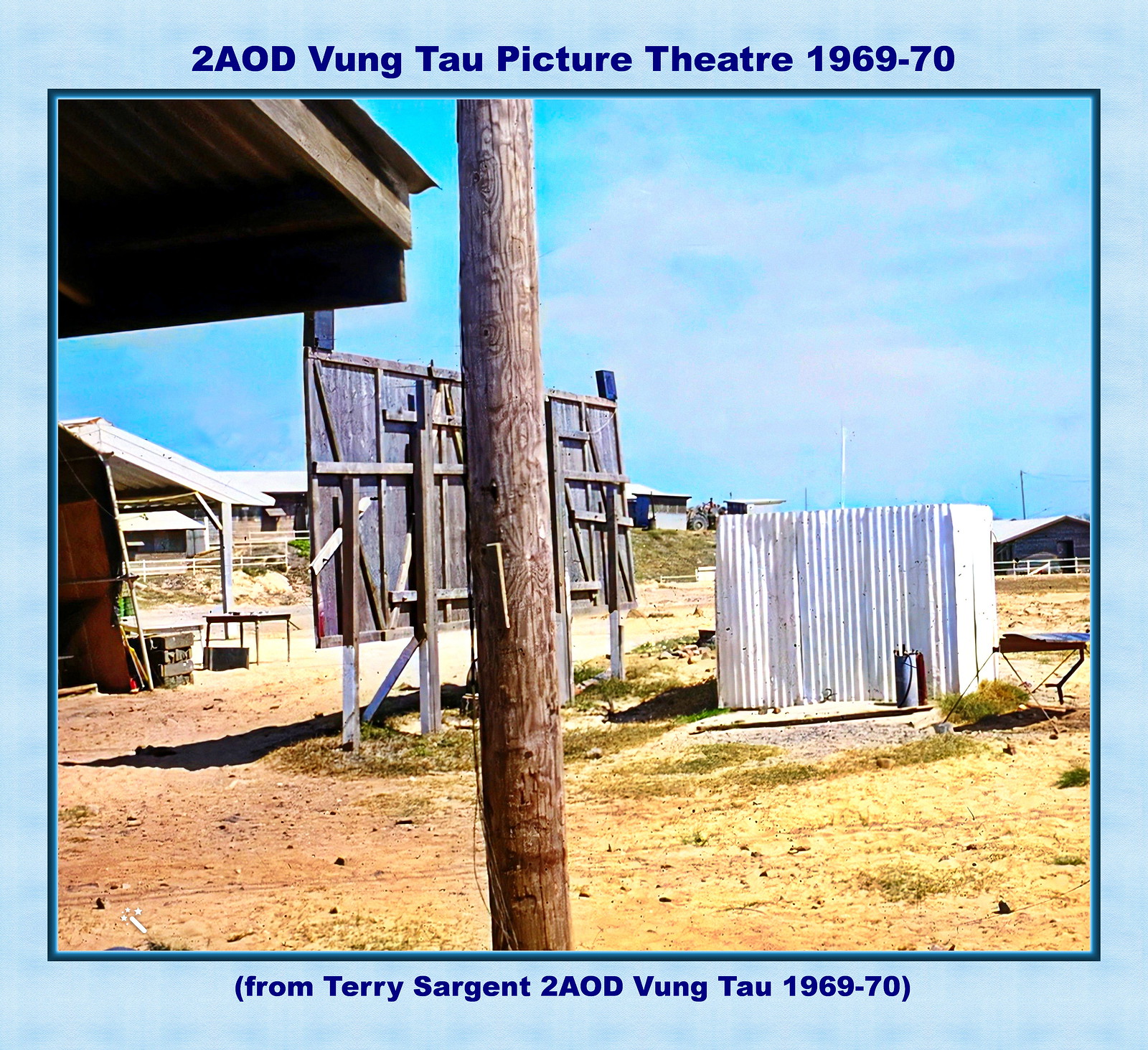This vintage photograph, taken in a war zone in Vietnam, depicts an outdoor theater in Vung Tau from 1969-70. The central focus is a projector screen constructed from plywood and two-by-fours, with a small white structure made from corrugated roofing material standing behind it. The ground is primarily dirt with patches of green grass. A prominent telephone pole rises in the center of the image, and to the right, there is a fenced-in square barrier made of metal. The background features buildings that resemble animal housing facilities, hinting at a farm or barn-like setting. An old table and a spray can are also visible. It is a sunny day, with blue skies dotted by puffy white clouds. The caption at the top of the image reads "2AOD Vung Tau Picture Theater 1969-70," while the bottom notes, "From Terry Sargent 2AOD Vung Tau 1969-70."